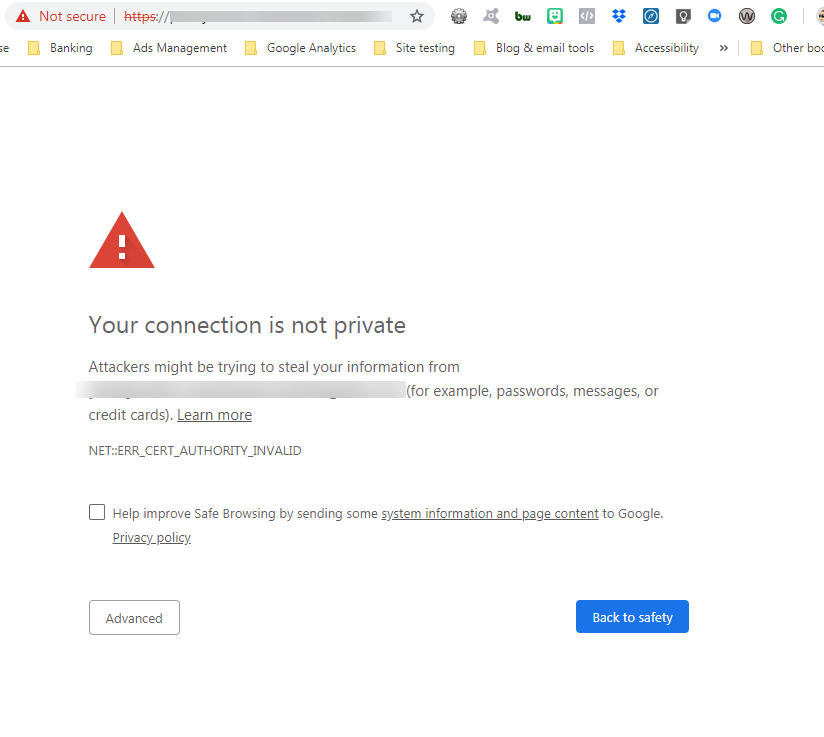Screenshot Description: 

The screenshot captures a web page featuring various elements indicative of a warning message. At the top, the address bar displays a "Not Secure" label in red on the left-hand side, followed by "HTTPS" also in red, crossed out by a diagonal line. The URL is obscured by a gray bar, making it unreadable. 

To the right of the address bar, a sequence of icons is visible: 
1. A gear icon
2. An unclear blob-like icon
3. The letters "BW"
4. A square with a smiley face
5. A gray square
6. Five triangles grouped together
7. A blue square
8. A gray square
9. A blue square possibly indicating recording functionality
10. A gray square with a "W"
11. A blue circle with the letter "G"

Below the address bar, there's a navigation menu with various selections including: 
1. Banking
2. Ads Management
3. Google Analytics
4. Site Testing
5. Blog and Email Tools
6. Accessibility
7. Other categories, abbreviated as "BO" with the remaining text obscured.

Prominently, a red triangle with a white exclamation point warns that "Your connection is not private," indicating potential security risks. The message elaborates that attackers might try to steal personal information like passwords, messages, or credit card details. 

A grayed-out example bar below the warning repeats the obscured address with the prompt for private data types. An underlined "Learn More" link follows, along with "Net::ERR_CERT_AUTHORITY_INVALID."

Further down, a checkbox invites users to help improve safe browsing by sending some system information and page content to Google, linked to the Privacy Policy.

At the bottom of the warning, there are two action buttons: 
1. A white button labeled "Advanced" on the left
2. A blue button labeled "Back to Safety" on the right.